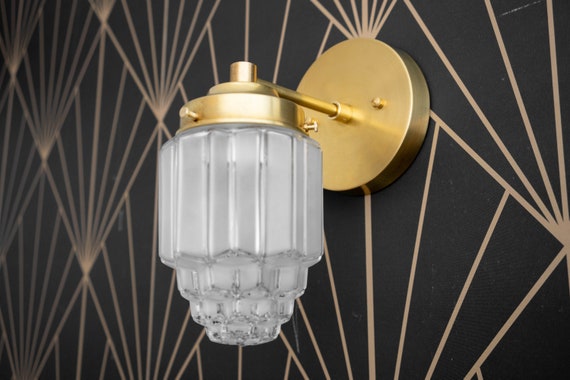The image depicts an elegant light fixture mounted on a wall, likely in a refined setting such as a hotel or upscale condominium. The wall is adorned with a sophisticated black wallpaper featuring an intricate geometric pattern: large diamond shapes outlined by gold lines, each containing five additional lines that radiate out symmetrically, resembling fans. This pattern repeats uniformly across the wall, creating a visually striking backdrop. The main focus of the image is the sconce, which consists of a gold circular base affixed to the wall with two visible screws. From this base, a slim gold rod extends outward, leading to a uniquely designed light fixture. The fixture itself resembles a miniature chandelier, composed of frosted glass shaped into a teardrop-like form with a wider base tapering downwards into a narrower extension. The overall aesthetic of the sconce and wallpaper combination exudes luxury and meticulous design.